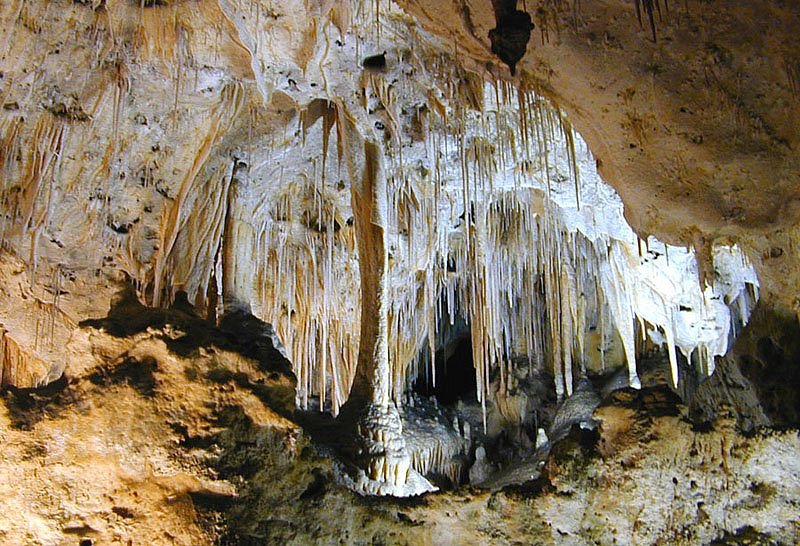The photograph captures the interior of a cave, showcasing formidable brown rock formations that dominate the space. Notable within the scene is a dark spot, possibly indicating the presence of a bat. The cave is adorned with striking stalactites and stalagmites; the stalactites, sharp and pointed, descend from the ceiling in a stark white contrast, while the stalagmites, heavier and thicker, rise from the cave floor. The rough-textured brown rocks are interspersed with patches of white, adding to the cave's rugged and raw aesthetic. Additionally, delicate water reflections can be observed at the cave's base, contributing to the natural and primeval atmosphere.